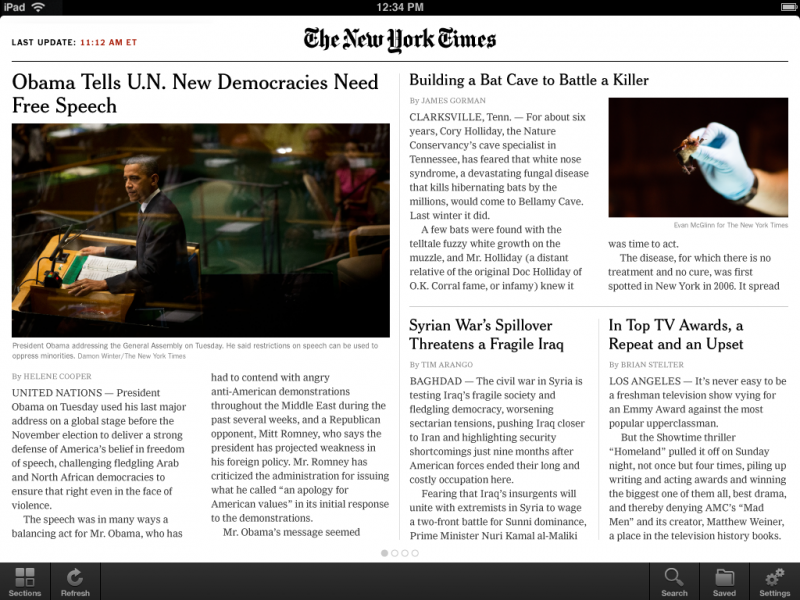**Caption:**

The image displays a digital interface with a predominantly black background. On the left side of the screen, in white text, it states that the iPad has a strong Wi-Fi connection. In the middle, the time is prominently displayed as 12:34 p.m. Over to the right, the battery icon in white indicates a full charge.

The background of the display changes to white, and on the left, in bold black letters, it reads "LAST UPDATE" with the time "11:12 a.m. ET" highlighted in red. Centered on the screen is the logo of "The New York Times," followed by a black line separator.

Below this, the content is divided into two sections. On the left side, it headlines an article titled, "Obama Tells New Democracies Need Free Speech," accompanied by an image of Barack Obama standing at a black podium. The text beneath reads: 

"By Helen Cooper. United Nations — President Obama on Tuesday used his last major address on the global stage before the November election to deliver a strong defense of America's belief in freedom of speech. He challenged fledgling Arab and North African democracies to ensure this right, even in the face of violence. The speech was, in many ways, a balancing act for Mr. Obama, who must contend with angry anti-American demonstrations throughout the Middle East in the past several weeks and Republican opponent Mitt Romney's criticism. Mr. Romney has accused the administration of projecting weakness in its foreign policy and issuing an 'apology for American values' in its initial response to the demonstrations. Mr. Obama's message seemed..."

The text is cut off at this point.

On the right side, there are titles of other news stories:
- "Building a Bat Cave to Battle a Killer"
- "Syrian War Spillover Threatens a Fragile Iraq"
- "Top TV Awards: A Repeat and an Upset"